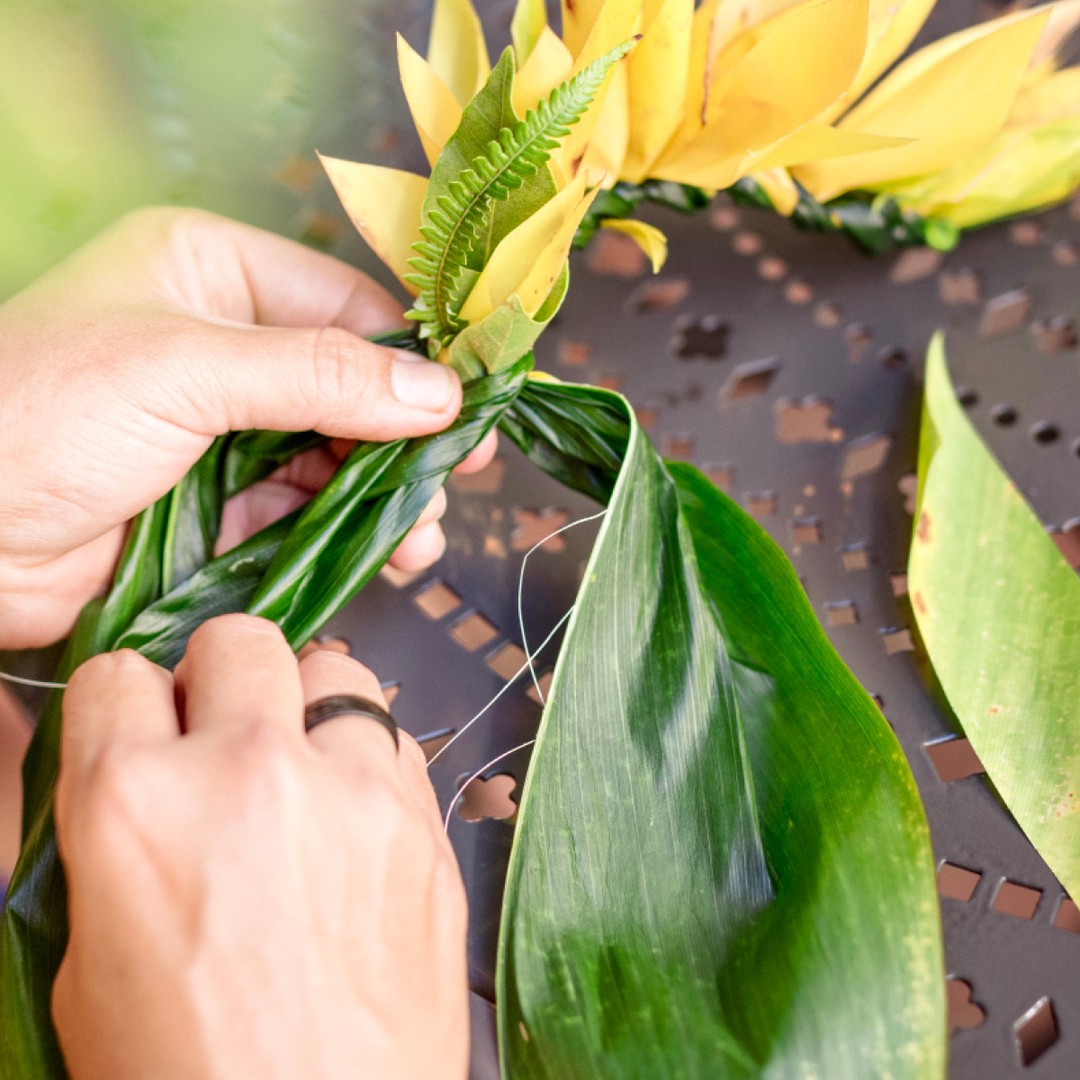This detailed color photograph captures a close-up view of a pair of human hands intricately working on a decorative arrangement using what appears to be a banana leaf and yellow blossoms. The hands belong to a white person, and the right hand is adorned with a dark brown, almost black, possibly wooden ring on the ring finger. The left hand firmly holds a bundle of ferns and leaves, with the thumb pressing into the center. The hands are skillfully twisting and tying the elements together with a thin white string, fashioning a braided or woven design. The arrangement features cascading rows of yellow blossoms extending from the knot. The work is being performed on a distinctive bronze-colored metal table characterized by various designing hole elements, including small squares, clubs, and diamonds. The left background of the image is notably blurred, drawing attention to the detailed craftsmanship in the foreground.